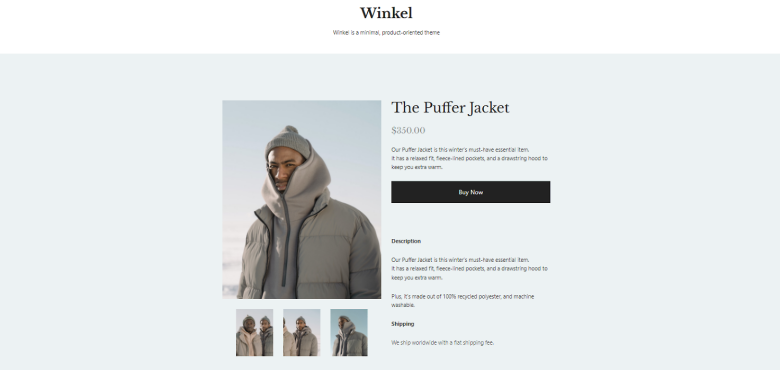The image features a clean design with a predominantly white background at the top. Centered in the middle of this white section, the word "Winkle" is prominently displayed in black. Below "Winkle," in much smaller text, it reads: "Winkle is a minimal, comma, broader-dash, oriented theme."

The background transitions into a light bluish-gray color. On the right side of the image, text in black reads "The Puffer Jacket" followed by a price of "$350.00." A descriptive paragraph follows, stating, "Our Puffer Jacket is this writer's must-have essential item. It features a relaxed fit, fleece-lined pockets, and a drawstring hood to keep you extra warm."

Below this paragraph, there's a black rectangular button with white text that says "Buy Now." Further down, there is a section titled "Description" in black. The description repeats, emphasizing that the Puffer Jacket is a must-have essential item and then adds, "Plus, it's made out of 100% recycled polyester and is machine washable."

Following this, a bolded title "Shipping" appears in black. The shipping section specifies, "We ship with a flat shipping fee."

The bottom part of the image showcases a large photo of a man wearing the described Puffer Jacket, which is gray in color and extends past his waist. He also wears a gray hat and has brown skin. Below this main photo are three smaller images, showing two different people wearing the same Puffer Jacket, providing multiple views of the product.